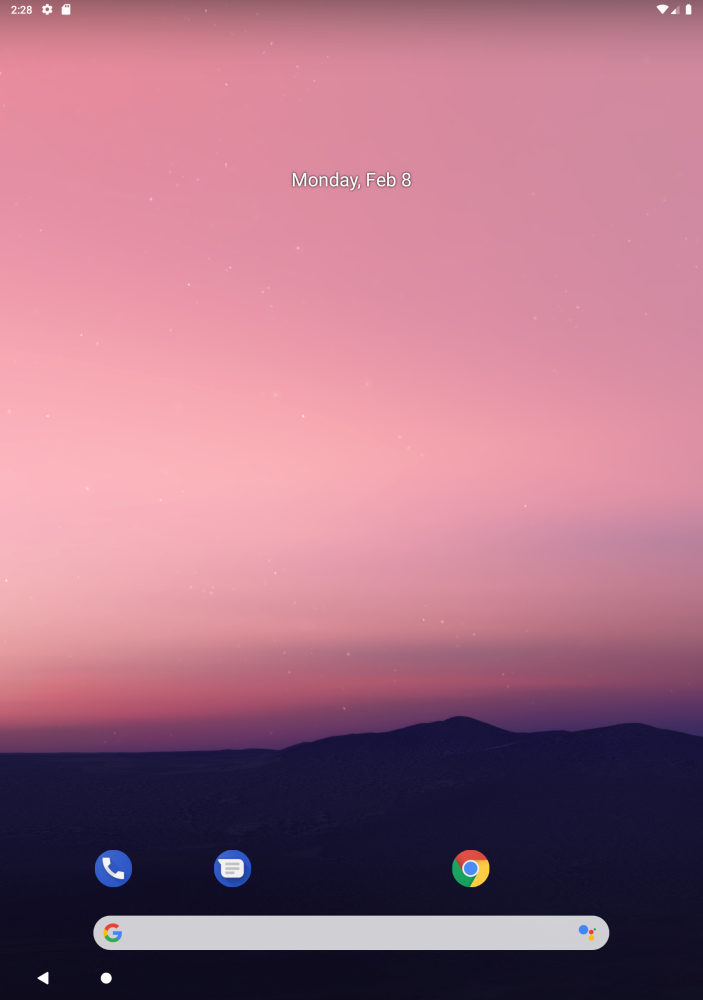The image appears to be a screenshot of a tablet's home screen. In the top left-hand corner, the time is displayed as "2:28" next to a small flower symbol and a slanted box with two holes at the top. On the right-hand side of the screen, the status indicators show that the device is connected to Wi-Fi, the battery is fully charged, and the network service is at half strength.

The background depicts a striking landscape featuring dark hills at the bottom, transitioning into a beautifully gradient sky. The sky starts with deep purples near the horizon, blending into darker pinks, and then light pinks towards the top. Scattered across the sky are small white dots resembling stars.

At the bottom of the screen, three horizontally-aligned app icons are visible: 
1. A blue circle with a white phone icon.
2. A blue circle with a text message icon.
3. The Google Chrome symbol.

Below these icons is a Google search bar, marked by a "G" logo and a solid gray bar. Additionally, at the very bottom left-hand corner, there's a white arrow pointing left within a small white circle.

Overall, the screen captures both functional elements of the device’s interface and the visually appealing background, offering a detailed overview of the tablet’s current display.